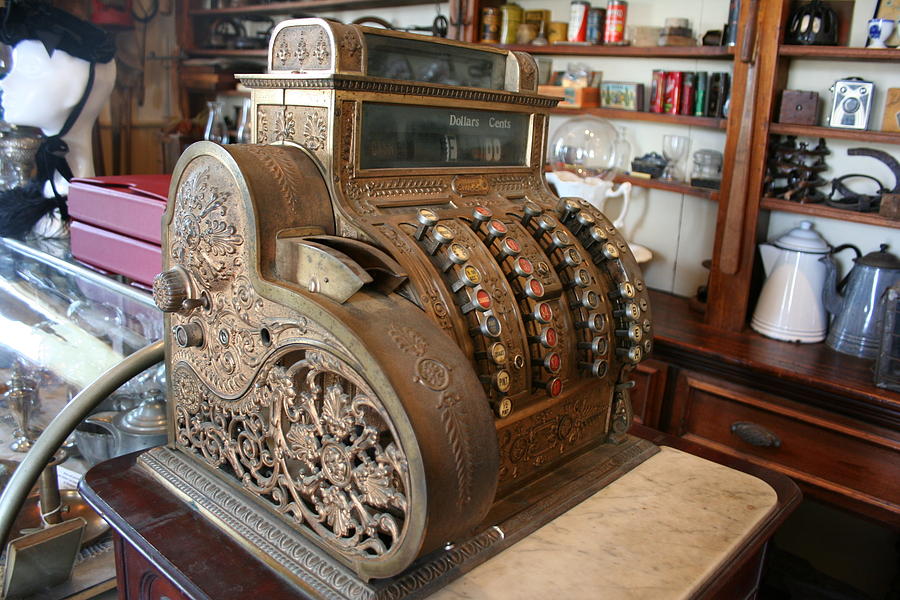The image showcases an ornate antique cash register, likely made of brass or bronze, adorned with elaborate decorative designs. The register features several rows of round buttons in colors like red, yellow, blue, and white, each with various letters and numbers inscribed. The top portion of the cash register has a display section indicating "dollars and cents" through analog rotating numbers. This grandiose and old-fashioned piece is set inside an antique shop, perched on a table or countertop.

Surrounding the cash register, the shop is brimming with vintage items including old teapots and kettles on wooden shelves, antique cans, silverware, and possibly a glass display case. In the background, white panel walls and colorful items on the shelves add to the antique ambiance. A mannequin head wearing a black hat tied under the chin is visible in the top left corner of the frame. Additionally, red books are noticeable behind the cash register. The scene captures a rich, historical atmosphere with various household collectibles enhancing the overall antique aesthetic.